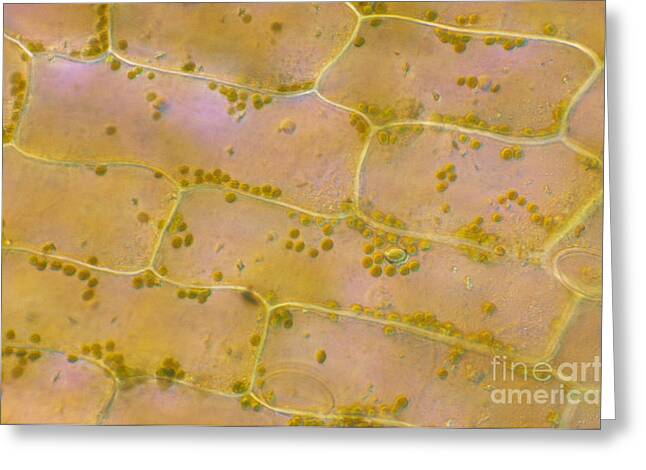This detailed image features the Fine Art America watermark in the bottom right corner, written in white lowercase letters on a beige background. The image depicts an intricate pattern of wavy, white lines that section off various areas filled with brown dots and specks. These dots are scattered throughout, some clustered together and some more isolated. The overall appearance of the background suggests an earthy beige color, with occasional blue hues adding a slight contrast. The photo's layout includes diagonal, almost rectangular shapes that intersect at different angles. The barren, reddish-brown ground might evoke imagery taken from an aerial perspective, possibly showing tree tops and shrubbery arranged in circular groupings, with yellow lines that could represent fence or property boundaries. This combination of microscopic and aerial elements creates an abstract and engaging visual narrative.